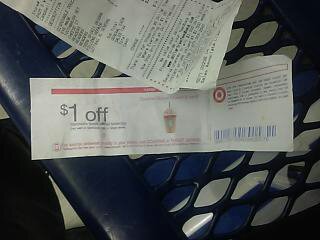The image features a Target coupon prominently displaying the retailer's recognizable logo. The coupon offers a discount of one dollar off a beverage, depicted with a straw. It rests on a black outdoor table with a perforated design. A partially visible receipt accompanies the coupon, though its origin is indiscernible from the visible portion. The right side of the coupon shows a scannable barcode for redemption at the store. The table is positioned on a gray concrete floor, visible through the table's holes.